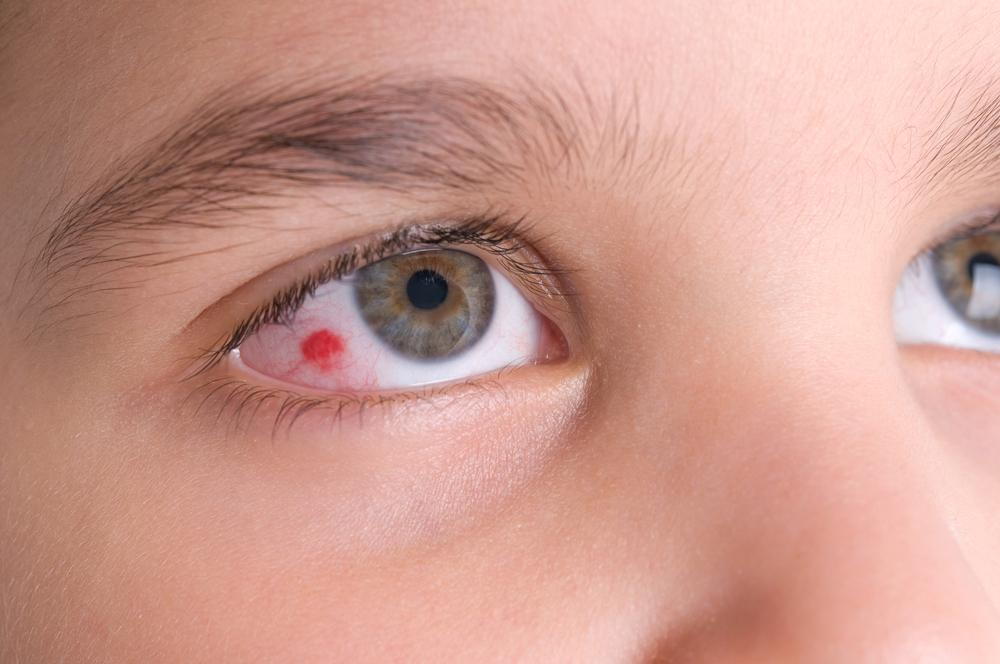This is a close-up photograph showcasing the eyes and the bridge of the nose of a young girl or woman. The primary focus is on the right eye, which displays a captivating hazel iris—an intriguing blend of blue and brown hues. The right eye also has a noticeable feature: a small red dot in the white area, indicating possible irritation or injury. Light brown eyebrows frame the eyes, with detailed individual hairs visible. The left eye is only partially seen, reflecting light and adding a touch of symmetry to the composition. Both pupils appear undilated, with the gaze directed upwards and to the right, suggesting an expression of concern or curiosity.